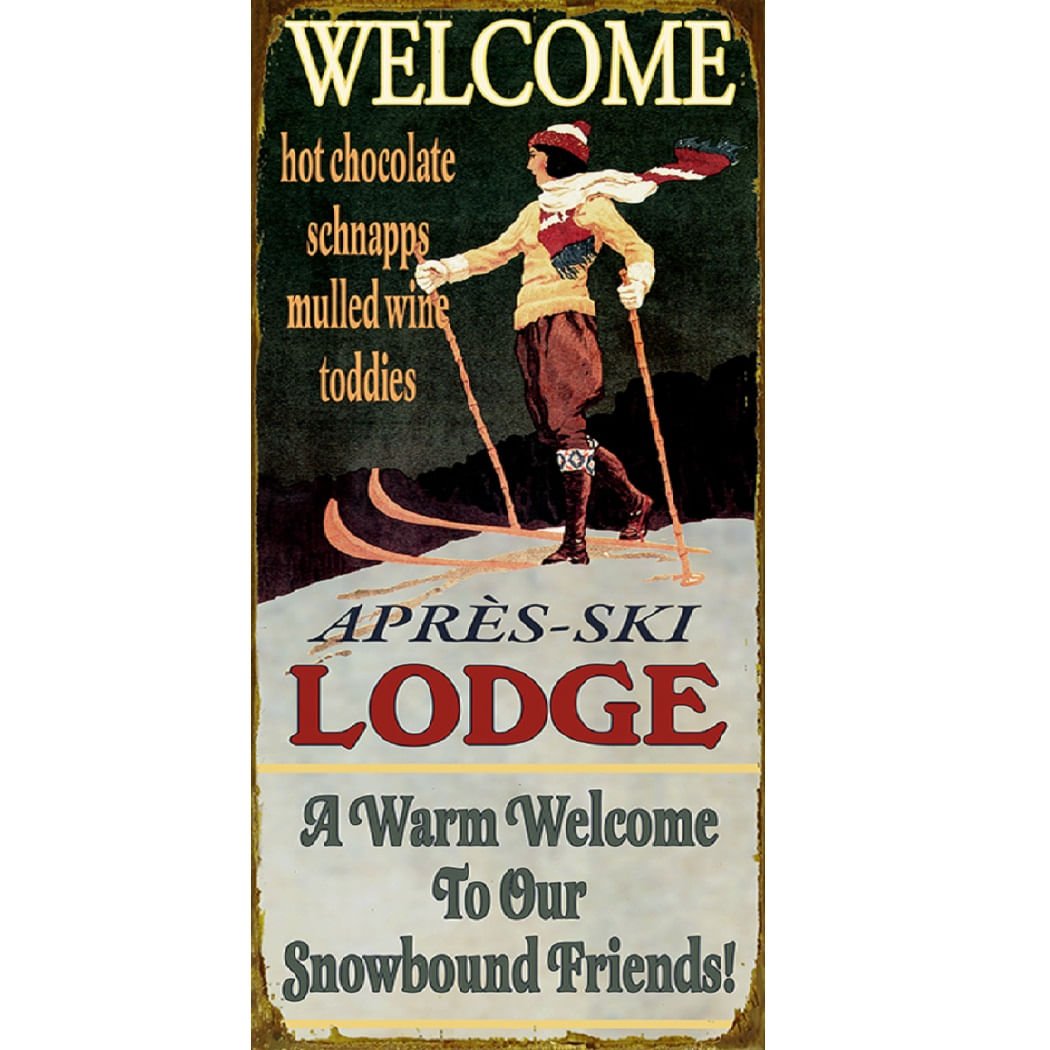The image is a detailed, color photograph of a vintage sign, likely made from metal with weathered, curling edges. At the top of the sign, the word "Welcome" is prominently displayed in white against a dark greenish-black background. Below this text, the central illustration features a woman cross-country skiing, evoking a nostalgic, old advertisement for a ski lodge. She wears old-fashioned, baggy brown pants, brown high-rise ski boots, a gold long-sleeve sweater, and a red and white knitted scarf adorned with green tassels at the ends. Her wooden skis and ski poles are a tan color. She also sports a red ski cap with a white stripe. 

The bottom portion of the sign mimics a snow-covered ground, adding to the vintage charm. Text on this snowy section reads: "Hot chocolate, schnapps, mulled wine, toddies, Apres Ski Lodge, a warm welcome to all our snowbound friends." The overall aesthetic of the sign suggests a welcoming, cozy ski lodge atmosphere, calling out to passersby with promises of warmth and comfort.